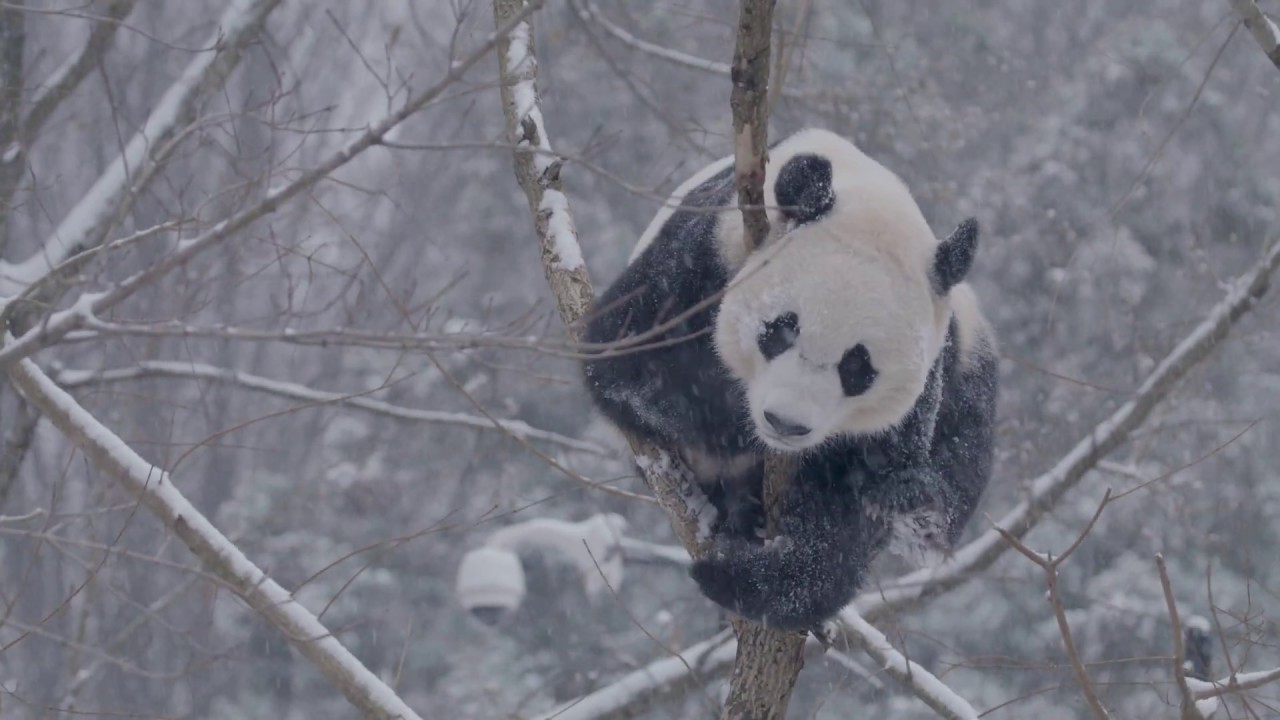In this unique color photograph, we see a snowy forest where all the leaves have shed off the trees. The ground and tree branches are blanketed in snow, emphasizing the cold, grim atmosphere. At the center, mid-right, a fully grown panda bear clings to a narrow, brown tree trunk. The panda, whose head is turned towards the viewer, showcases the iconic black and white markings: black ears, round black patches around its eyes, a black nose, black legs, and a predominantly white head and upper body. Snowflakes drift through the air, adding to the wintry scene, and snow has also settled on the panda itself. Behind the panda, a lamp post, or what could be a surveillance camera on a post, is visible beneath the tree branches, hinting at a possibly urban setting. The overcast sky, combined with the snow-covered trees and a distant hill, creates a stark yet striking backdrop for this compelling image.